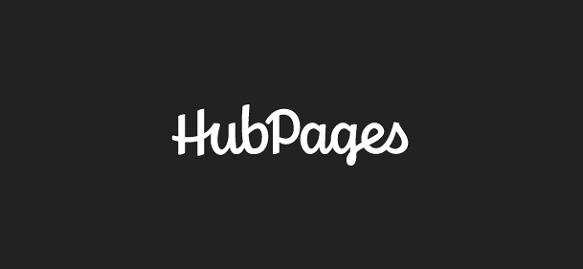The image features a predominantly black rectangle as its background, providing a stark contrast to the text situated at its center. Written in an elegant white cursive font, the words "Hub Pages" stand out prominently, with the 'H' and 'P' capitalized while the rest of the letters remain in lowercase. The design is reminiscent of the playful, whimsical aesthetic often associated with cupcake decorations, thanks to the flowing, artistic style of the font. Surrounding the central text is a considerable amount of empty space, which further draws attention to the minimalist and uncluttered nature of the design. Beneath the black rectangle, a larger expanse of plain white space exists, devoid of any additional elements or details.